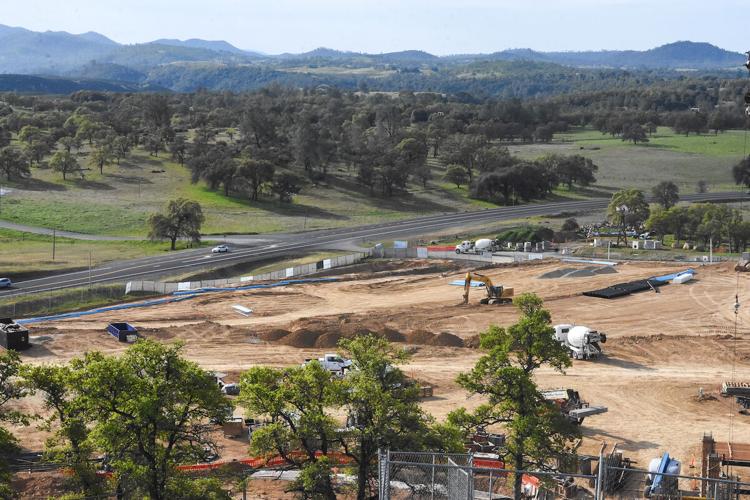This panoramic photograph, likely captured from a drone or taken from six or seven stories up, depicts a vast construction site set amidst a countryside landscape. The focal point of the image is the expansive construction area in the foreground, which is enclosed by a metal chain-link fence. This site is characterized by large dirt mounds and active machinery, including a digger and a cement truck with a prominent cylinder on its back. Several other vehicles, such as a truck and a white pickup truck, are also present within the fenced area.

In the lower center of the image, another cement truck is visible, suggesting road construction activities. The foreground includes trees to the left. The photograph appears split by a major highway running horizontally through the middle, featuring at least four lanes with several cars on it.

Beyond the highway lies a natural landscape dominated by dense green trees and a smaller road that branches off to the right. The far background is graced with a hazy blue sky and a scenic mountain or hill range, covered in lush greenery. There are no signs of buildings or houses, emphasizing the rural setting of the construction site.